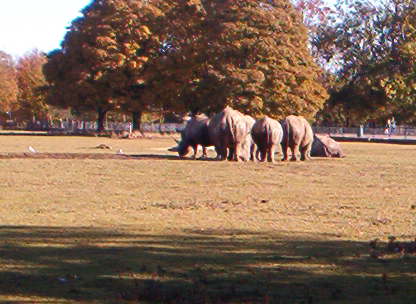This small, rectangular, and horizontal color photograph captures a serene scene of a small herd of rhinoceroses in a wildlife park, characterized by North American foliage suggesting it is autumn. We observe the rear ends of three rhinos: one lying down on the right, another grazing on the left, slightly turned and silhouetted in shadow, and their tails facing us. The ground is a mix of dry, brownish-green grass interspersed with dead plant matter. Large deciduous trees with yellowish and orangey leaves in the background cast shadows across the scene. In the far right-hand frame, a couple of tiny figures—some people—are visible, emphasizing the park setting, along with a faint outline of a low chain-link fence. Additionally, a couple of small white birds dot the ground near the rhinos, which further enhances the wildlife habitat atmosphere. The overall snapshot has an informal quality, indicating it wasn't professionally taken.